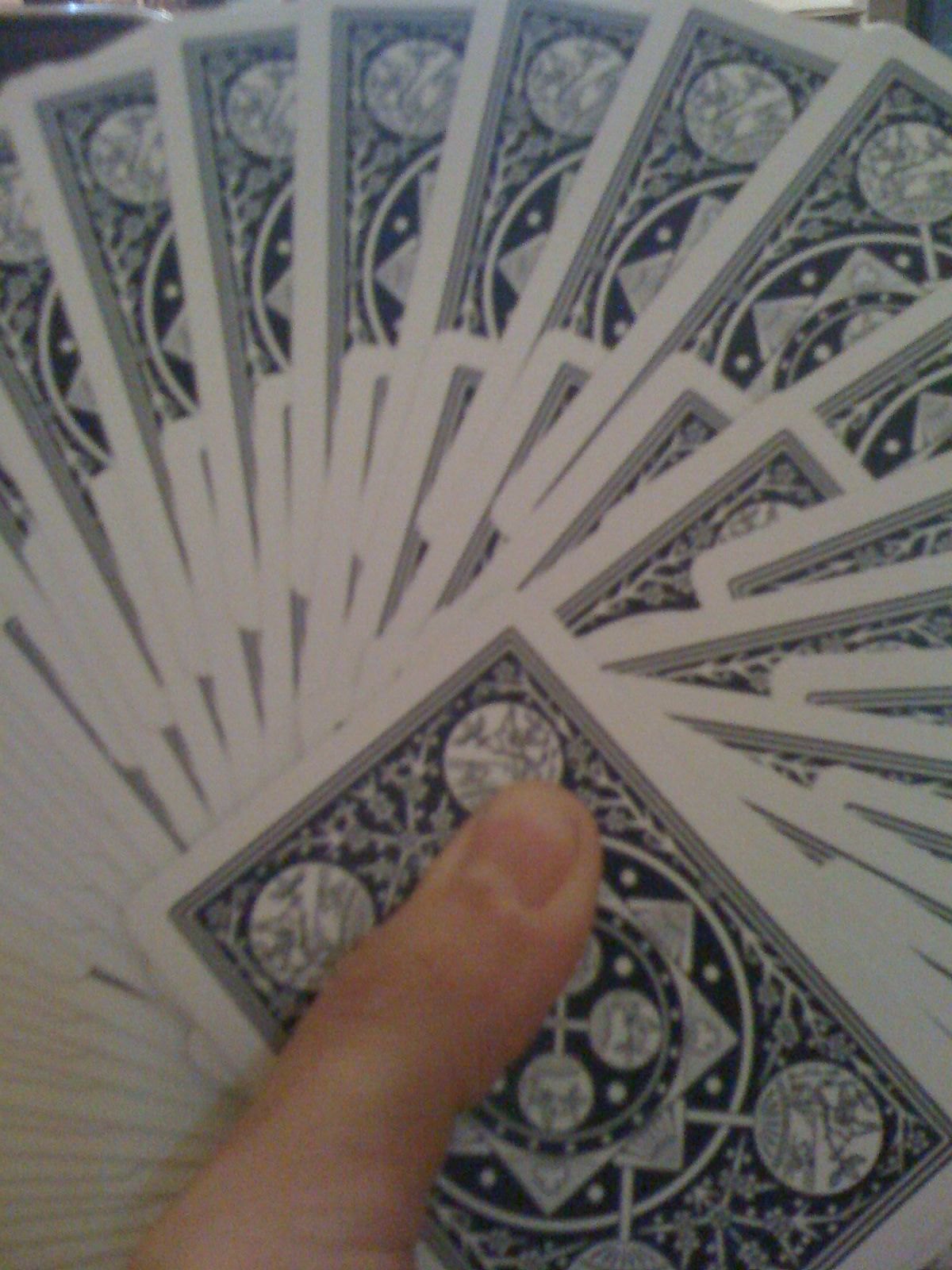The image displays a close-up of a thumb, presumably belonging to a white male, holding a meticulously fanned-out set of playing cards. The thumb is positioned at the bottom left of the frame, securely gripping the cards, which are evenly spaced and arranged in an elegant fan shape. Some of the cards are oriented away from the holder, while others are aligned horizontally. The skin of the thumb appears smooth with minimal wrinkles, and it has a pinkish hue with a white edge near the hand. The cards themselves are blue, contributing to the overall aesthetic of precision and skill in the display.